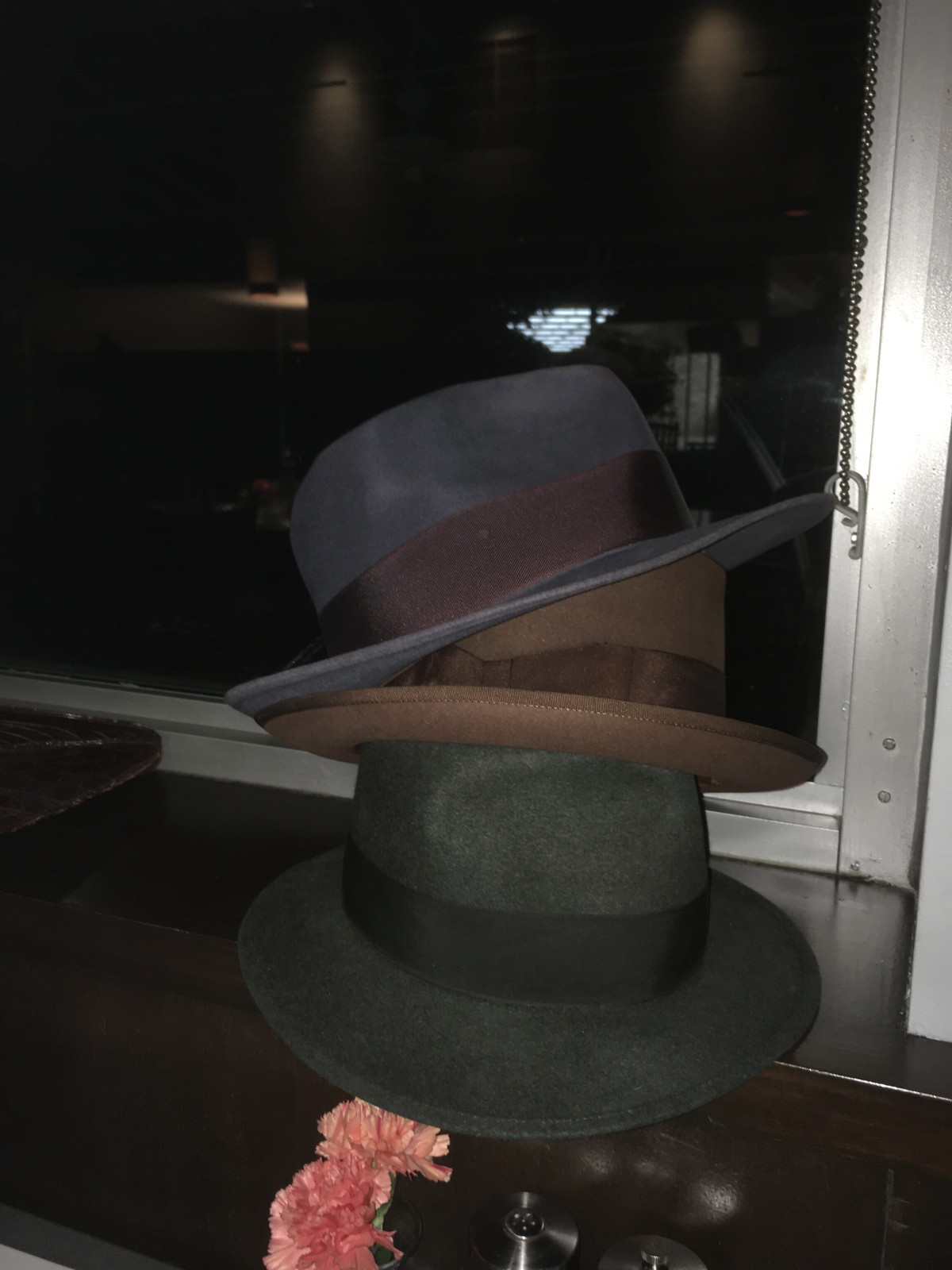In the image, three fedora-style hats are stacked atop one another on a dark wooden windowsill framed with chrome-colored steel. The bottom hat is a dark green with a matching dark green band. Above it, there is a medium brown fedora, slightly tilted back, featuring a darker brown band. The top hat, angled with the left side lower than the right, is medium gray with a purplish-gray band. The scene is set against a silver-framed window, beyond which it is dark, preventing any view outside. In front of the stacked hats, two pink carnation flowers are visible, with a bit of their green stems showing, adding a touch of color to the composition. To the right side of the window hangs a chain, contributing to the intricate details of the setting.